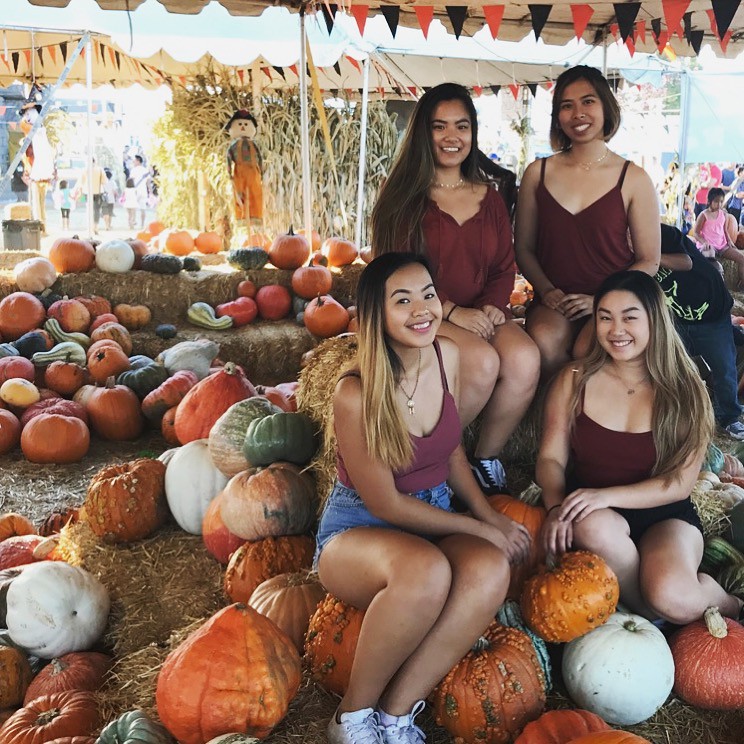This photograph captures a joyful moment of four teenaged Asian girls sitting amidst an abundance of pumpkins and gourds of various colors, including white, light orange, deep orange, green, with some displaying stripes, and yellow. The girls, all smiling warmly at the camera, are dressed similarly in maroon tank tops and shorts, exhibiting different hair styles; two at the front feature long, dark hair with blonde streaks, while the two at the back have long and slightly shorter dark hair respectively. They sit in what appears to be an open tent or canopy, perhaps at a fair. The festive setting is decorated with bales of hay, a scarecrow, and bunting of orange and black triangles, suggesting a Halloween or fall theme. The scene is bustling with activity as hinted by the crowds in the background, adding to the lively fair atmosphere. Far to the top right, a small girl with dark hair in a pink vest top can also be seen, adding a touch of charm to the snapshot.